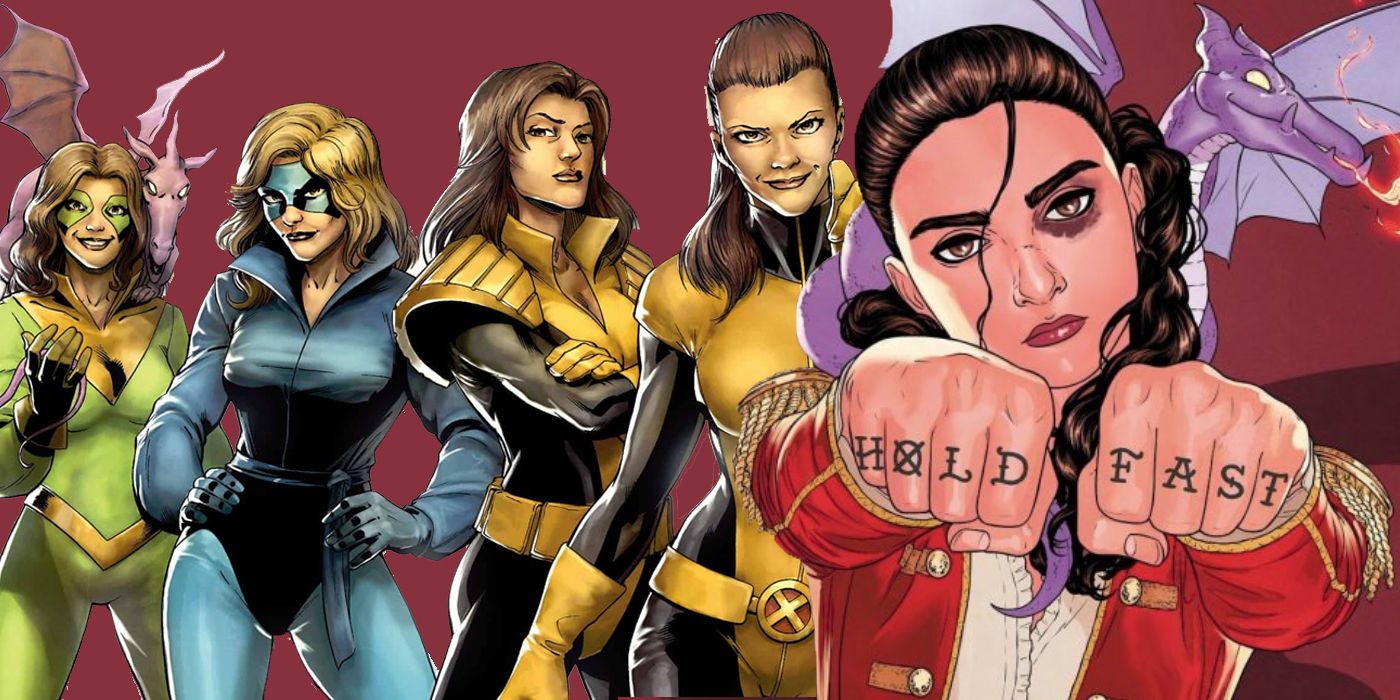This vibrant comic book illustration showcases a lineup of five distinct female superheroes against a reddish-purple background. Starting from the left: the first heroine is clad in a tight green bodysuit with gold accents and wears a green mask over her eyes. She has long brown hair and a mischievous purple dragon perched on her shoulders, smiling warmly at the viewer. Next to her, a woman in a shiny blue jumpsuit with a high collar and matching sash exudes confidence. She sports a blue mask that covers the upper half of her face and has shoulder-length blonde hair. Moving further right is a third woman in a sleek black jumpsuit adorned with a prominent yellow belt, shoulder pads, and a high collar. She has long brown hair and looks down at the viewer with her arms folded. Adjacent to her is another brunette superhero wearing a striking combination of black and yellow, including yellow gloves and a bathing suit over her rubber bodysuit, smiling directly at the audience. On the far right stands a young girl in a red jacket and white undershirt, her brown hair pulled back into a ponytail. She holds her fists up to the camera, showcasing "HOLD FAST" tattooed across her knuckles, with a small purple dragon perched on her shoulder. Both she and the dragon maintain a stern gaze towards the viewer.